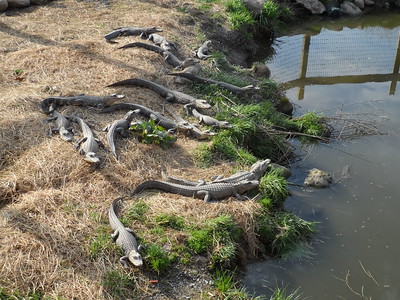This color photograph depicts a muddy, murky body of water bordered by a bank where approximately 10 to 15 small, grayish alligators or crocodiles are scattered haphazardly. The view appears to be taken from above at an angle, capturing both the river and the grass-covered embankment. While most of the grass is burnt, brown, and yellowing, a few green tufts remain near the water's edge. The water itself is muddy olive green, filled with rocks, twigs, and debris. The alligators, with their long tails and scaly skin, are either lying near each other or more spread out, with some seemingly crawling towards the water. At the top of the picture, a faint reflection of a fence suggests that these reptiles might be within an enclosed area.